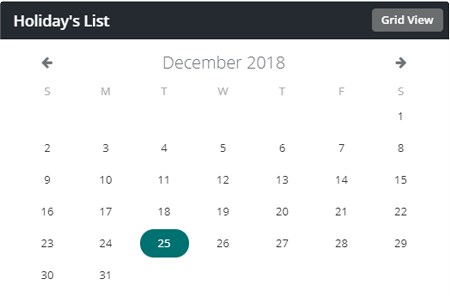The screenshot depicts a calendar app with a dark gray header at the top. The header features the text "Holidays List" in white on the left side and a light gray rectangular button labeled "Grid View" on the right. Directly beneath the header, there are left and right arrows in gray on either side of the displayed date "December 2018." Below the date, the days of the week are denoted by their initial letters (S, M, T, W, T, F, S) in light text. The numerical days of the month follow, starting with '1' under the first Saturday and ending with '31' under the last Monday, arranged in a grid format without visible borders or lines and displayed in light gray text. Notably, December 25th, which marks Christmas, is highlighted with a teal, capsule-shaped background and white text, distinguishing it from other days in the calendar. The month spans six weeks, as indicated by the arrangement of the days in the grid.